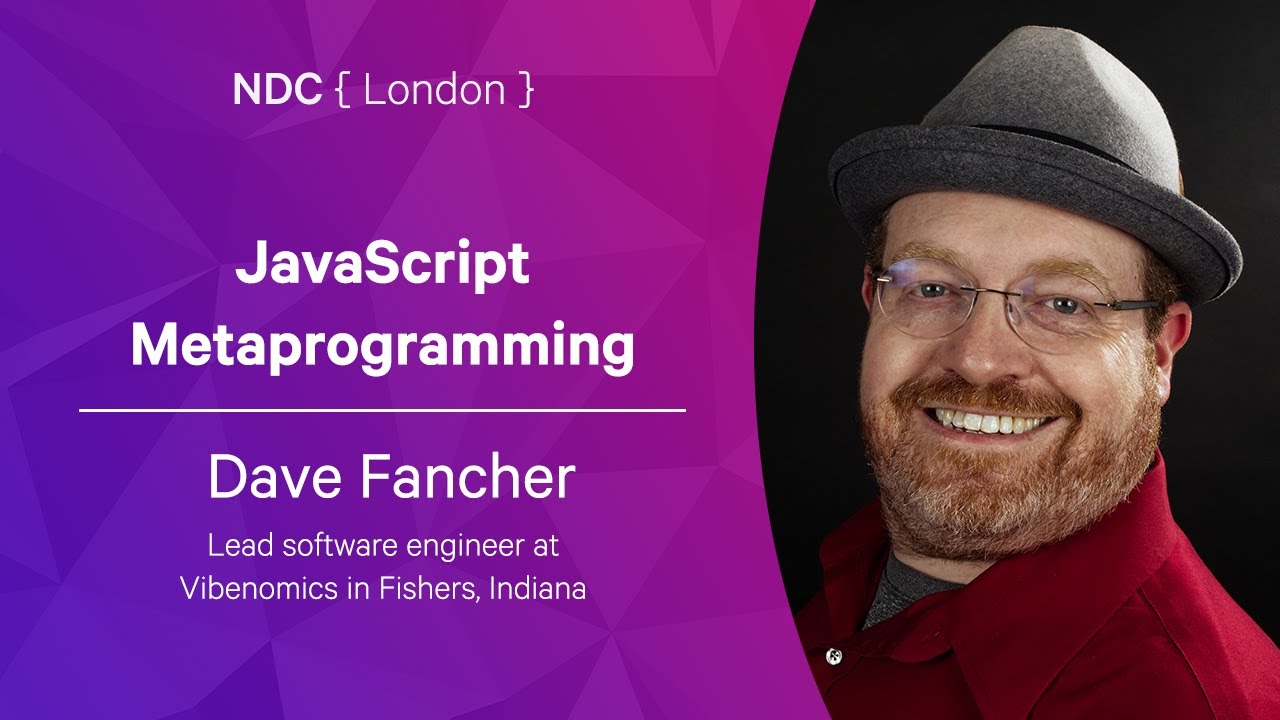This image captures a computer screen displaying a vibrant and colorful backdrop. The left side of the screen is dominated by a rich purple hue, seamlessly transitioning into a fuchsia or bright pink shade as it moves towards the right. Positioned on the far right, there is a photo of a man adorned in a stylish dress hat and clear glasses. He sports an auburn mustache paired with a beard that sprinkled with strands of gray or white. The man is dressed in a red shirt layered over a gray t-shirt, and his face beams with a broad, cheerful smile.

Overlaying the gradient background, in the upper left corner, the text "NDC [London]" is prominently displayed. Moving towards the center, the screen shows the title "JavaScript Metaprogramming" in bold letters. Below a separating white line, the name "Dave Fancher" is listed, followed by "Lead Software Engineer at Live Non X in Fishers, Indiana" in smaller font, providing details about the speaker. This composition suggests a professional presentation slide, likely for a tech conference or webinar.